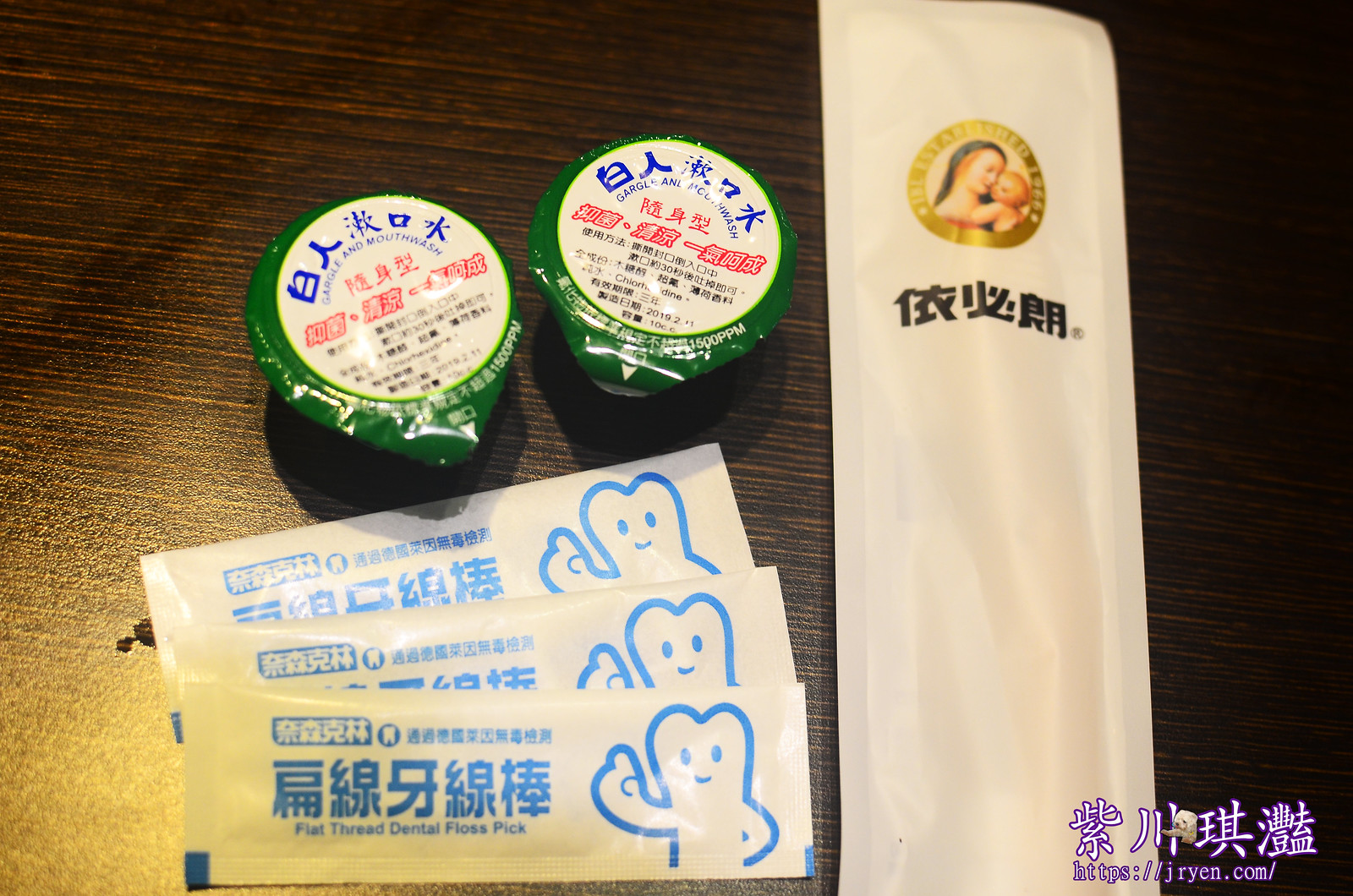The photograph depicts several items arranged on a dark brown wooden table with visible horizontal stripes. In the lower right-hand corner, there is a URL, "http://jryen.com/", written beneath Japanese text in purple, accompanied by a small image of a dog's head with arms. The image prominently features two circular sauce packets with blue and red Japanese text on a dark green background, and three rectangular white sachets labeled in both Japanese and English with "flat thread dental floss pick." Each sachet also has a blue cartoon character resembling a tooth with arms. Additionally, a long rectangular white package stands out with black Japanese text and a circular emblem featuring a light-skinned woman with golden hair, adorned in a dark blue cloth scarf, holding a blonde-haired baby, suggesting a depiction of the Virgin Mary and baby Jesus. The overall scene combines various text and images, melding both practical items and religious iconography, all set against a richly textured wooden surface.